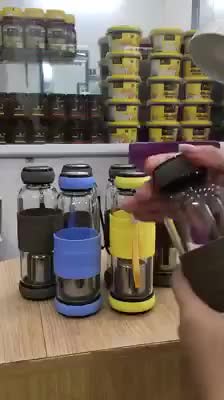The image depicts a wooden table adorned with several water bottles, all sharing a similar cylindrical, glass design but differing in color and details. At the forefront, there are two noticeable bottles: one with a blue lid and cover, and another with a yellow lid and cover, both sitting beside three bottles that feature black accents. Each bottle appears to have a metallic, cylindrical component at the bottom. On the right side of the image, a pair of hands can be seen holding what is likely a black water bottle, though the image is grainy and somewhat blurry, making it hard to discern the exact object held. In the background, there is a shelf with stacked tubs on the left side and a collection of shorter bottles, some with yellow lids, on the upper shelf in the left-hand corner. The shelf displays an array of black, brown, and yellow objects, set against a backdrop of white walls.